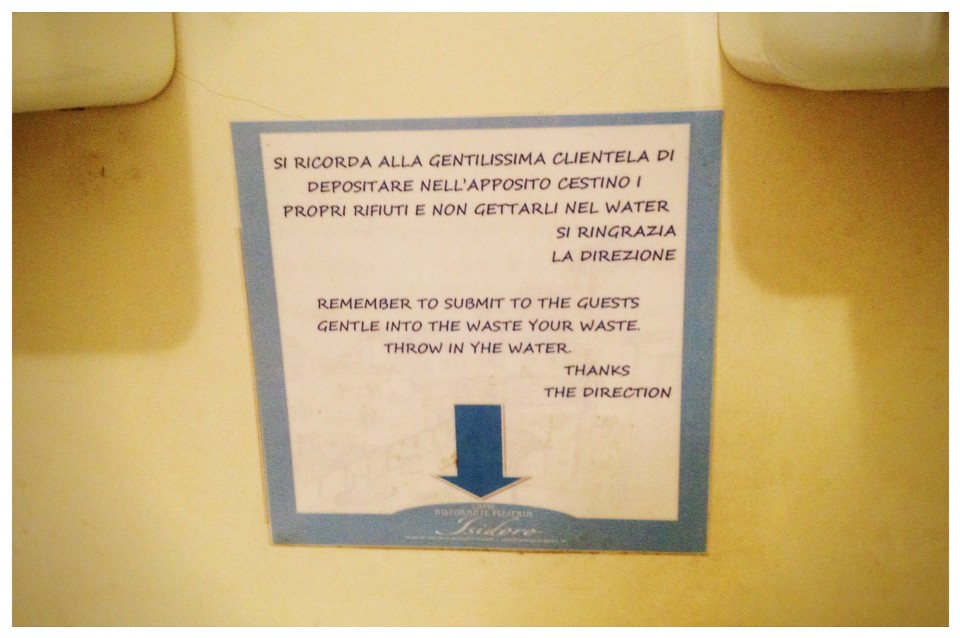The image depicts a sign posted on a yellowish-tan wall, possibly in a hotel bathroom. The sign is bordered with blue and contains text in both Italian and English. The English portion reads, "Remember to submit to the guests. Gentle into the waste. Your waste. Throw in the water. Thanks the direction," indicating instructions for waste disposal, likely in a restroom. The text is confusing, hinting that the sign might have been poorly translated. The sign also features a blue downward-pointing arrow. The wall shows signs of dirt, and there are two white fixtures at the top of the image, which appear to be bathroom sinks.